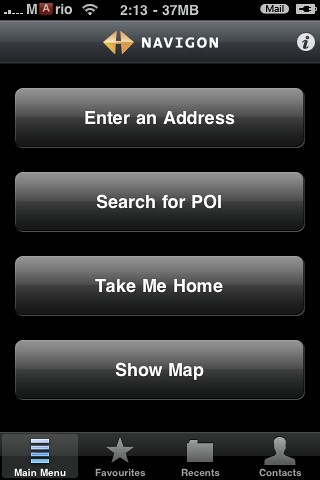This image is a detailed screenshot from a mobile device displaying the main menu of the Navigon navigation app. At the top, a gradient gray banner features the app's name "Navigon" in white letters with a gold logo beside it. The smartphone's status bar shows the signal strength and time above this banner. Below the banner, four touch-activated buttons appear in light gray with white text: "Enter an address," "Search for POI," "Take me home," and "Show map." Beneath these buttons is a row of icons for additional navigation within the app, starting from the left: "Main Menu," "Favorites" marked by a star, "Recents" indicated by a file folder icon, and "Contacts" represented by a humanoid figure. The background of the entire screenshot is a varying shade of black, enhancing the contrast and readability of the interface elements.